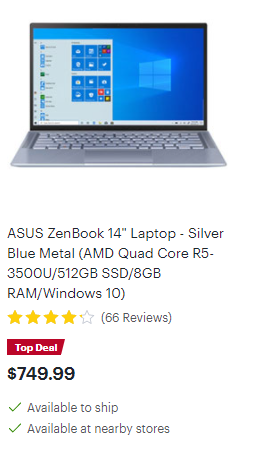The image depicts a web page designed for purchasing products, prominently showcasing a specific laptop computer. The background of the web page is white, ensuring that the featured product stands out clearly. Positioned at the top is a photograph of the ASUS ZenBook 14-inch laptop. The laptop's screen displays a blue background with the Windows logo on the right side, and the screen itself is outlined in black, which matches the sleek black edges of the actual laptop. The keyboard of the laptop is entirely gray, providing a stylish contrast to the darker screen border.

Beneath the product image, there is a detailed description. The text, in black, reads: "ASUS ZenBook 14-inch laptop, silver blue metal, AMD quad-core R5 3500U, 512GB SSD, 8GB RAM, Windows 10." Below this description, the product has been rated 4 out of 5 stars, based on 66 customer reviews. The price of the laptop is prominently displayed underneath the rating, listed as $749.99.